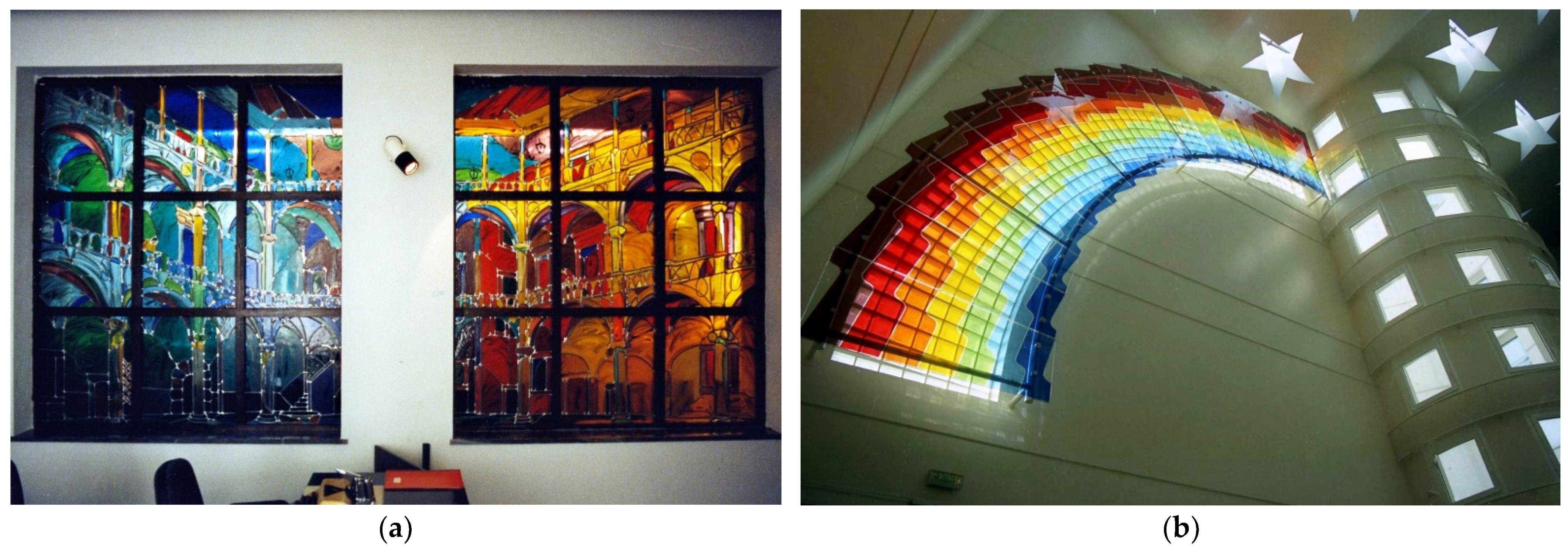The image consists of two side-by-side rectangular images labeled "A" and "B." 

Image A features two stained glass windows, each with a 3x3 grid of panes, framed in black. The windows exhibit a variety of colors, from deep blues and oranges to bright whites, yellows, reds, greens, and purples. The stained glass forms a picturesque scene reminiscent of architectural landmarks like the Colosseum, with one side showcasing brighter hues and the other a palette of darker shades such as dark red, brown, tan, and purple.

Image B portrays a stunning stained glass artwork designed in a zigzag pattern, evoking the vibrant spectrum of a rainbow. Dominated by colors like purple, red, orange, yellow, green, light blue, and dark blue, this artwork is accentuated by white star motifs. The backdrop is a white wall adorned with numerous small, square windows and star decorations, enhancing the overall ethereal effect of the rainbow glass design.

Both images exude a captivating interplay of light and color, evoking a sense of whimsical artistry and architectural beauty.